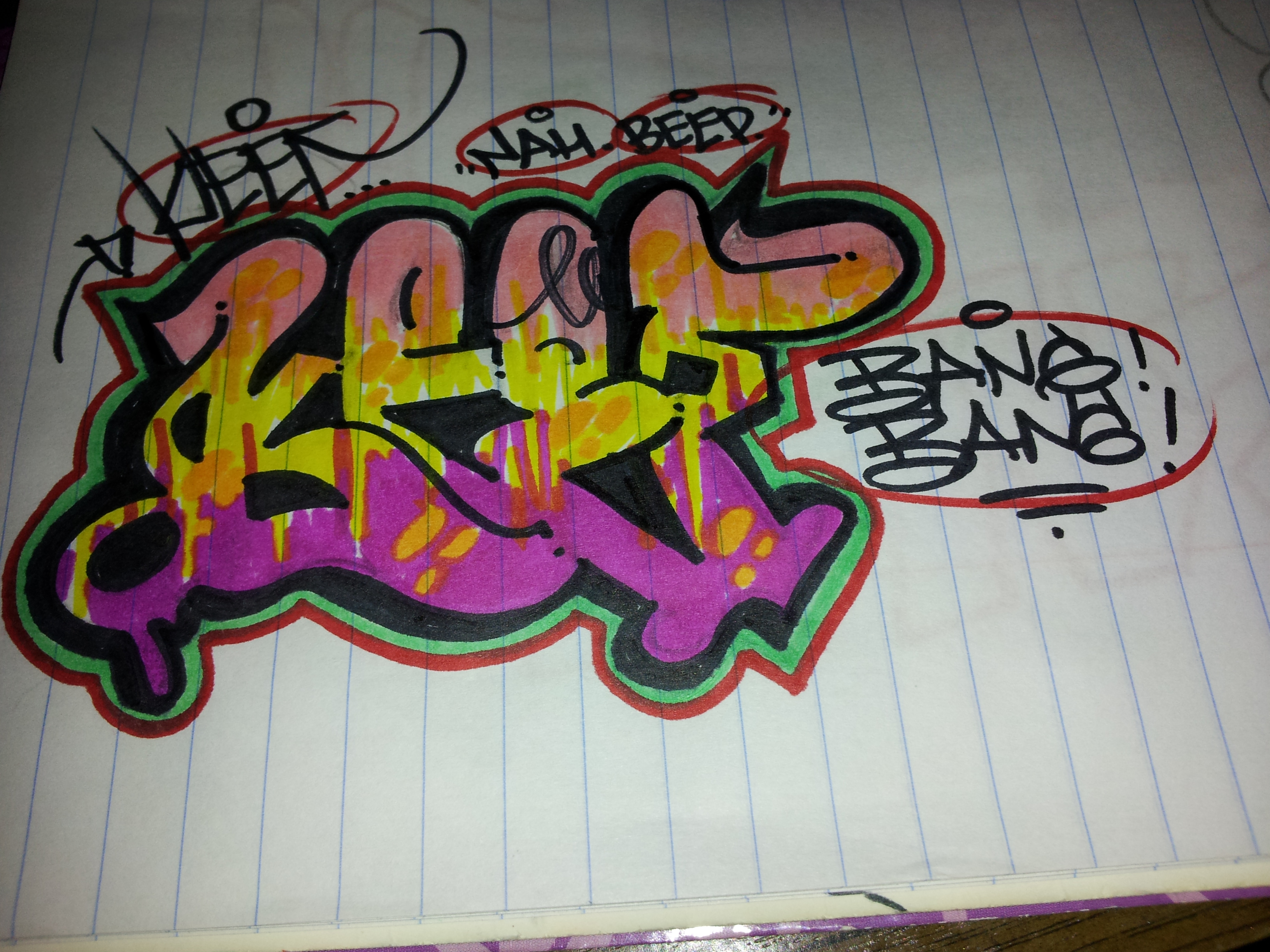The image features graffiti-like art drawn on lined notebook paper, likely positioned on a dark-colored table illuminated by a slight shine. The edge of the notebook appears to be purple. Central to the image is a large, colorful tag featuring swirls of pink, yellow, and purple that bleed into each other, creating a rainbow-like effect. This tag is outlined successively in black, green, and red. To the right of this vibrant tag, the words "Bang Bang" are handwritten in black and underlined, encased in a red speech bubble. Above the central tag, there are additional words: "Knob Beep" circled in red and written in black, and other writings in blue, identified as “beep,” “nah,” and possibly “peak.” Additionally, on the left side of the image, there is more text in black, written in an urban or gangster style, but it remains largely illegible. The intricate details and layered colors create a dynamic piece against the structured background of the notebook paper.